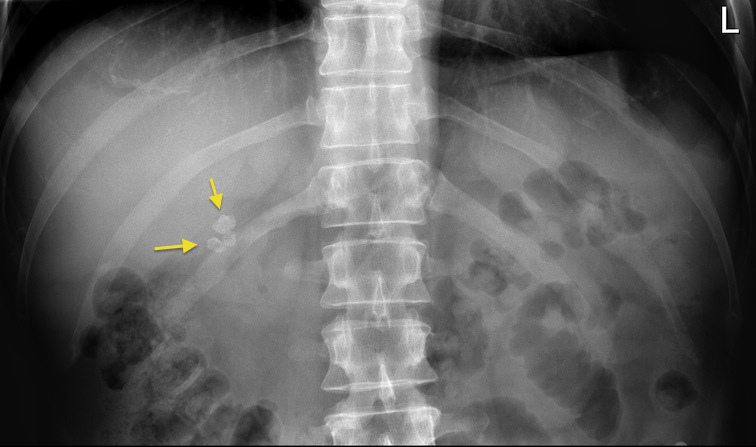This detailed image is a black and white radiographic x-ray scan in landscape orientation, showcasing the upper torso of a patient. Central to the image is the spine, with clearly visible vertebrae in a light white hue. Semicircular rib structures extend from both sides of the spinal column. On the left portion of the scan, the image highlights a small white mass or masses near the ribs, indicated by two yellow arrows—one pointing from above and the other from the left. Additionally, a white "L" in the top right corner marks the left side of the body. The x-ray captures both lighter and darker splotches with no explanatory text accompanying them, leaving the specific nature of these irregularities open to interpretation.